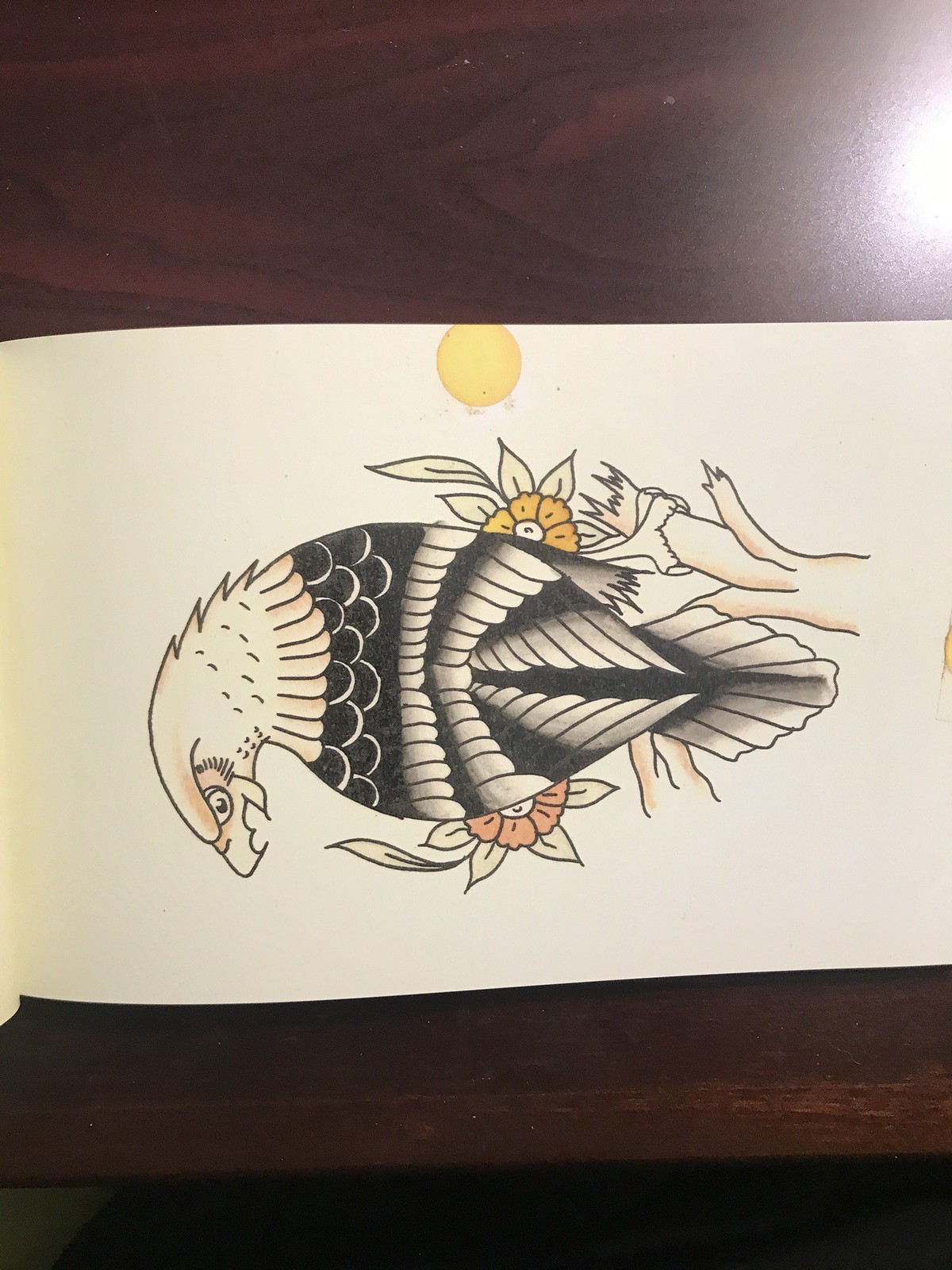This photograph captures a detailed drawing of an eagle, positioned slightly askew on a white sheet of paper bound within a book. The fold of the book is visible on the left side, indicating its presence on a dark, cherry-colored wooden surface. The eagle, distinguished by its white head, curved beak, and intense dark eyes, is a focal point of the artwork. Its wings feature an alternating pattern of black and white feathers, creating a striking visual effect. The tail feathers are predominantly black, with white tips adding contrast. The majestic bird perches gracefully on a brown wooden branch, partially obscured by blooming flowers. To the right of the drawing, a circular tan-colored stain marks the page, adding a touch of imperfection to this otherwise meticulous composition.